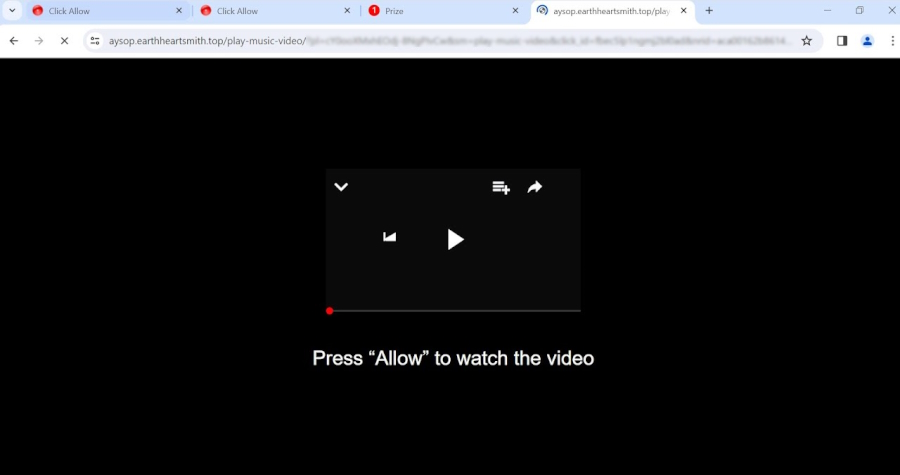This image appears to be a screenshot of a website with various UI elements. Here's a detailed caption describing the image:

---

The image is a screenshot from a website that features multiple design elements arranged within a layered border structure. The outermost border, about an inch in thickness, is light blue, followed by an inch-wide white border, and the remainder of the background is black.

In the top left section of the light blue border, there's a small, black greater-than sign (>), oriented to point downward. To the right, within the blue border, is a small red circle containing black text that reads "click allow." This circle is followed by approximately an inch of space and a black 'X'. A vertical line divides this section from another red circle labeled "click allow" alongside another black 'X'. Another vertical line separates this part from a white circle with text "prize" and yet another black 'X'.

The next section features a lit-up white area containing a blue circle with black text stating "AYSOP.EARTHHARTSMITH.TOP\PLA," followed by another black 'X'. Transitioning back to the light blue border, there’s a black plus sign on the left, a black 'X' next to it, and a black square adjacent to them. The right side of this arrangement includes a black minus sign. In the white portion below, there's a left-pointing black arrow, a grey right-pointing arrow, a black 'X', and a partially obscured search bar. On the extreme right, there are three black vertical dots, a blue circle with a profile icon, and a lighter black area in the center.

At the center, this lighter black portion hosts a downward-pointing white greater-than sign in the top left corner, a list icon, and a share icon on the right. A horizontal play bar rests at the center, featuring half of a rewind button on the left side. In the bottom left corner, a small red dot appears with the text "press (allow) to watch the video" underneath.

---